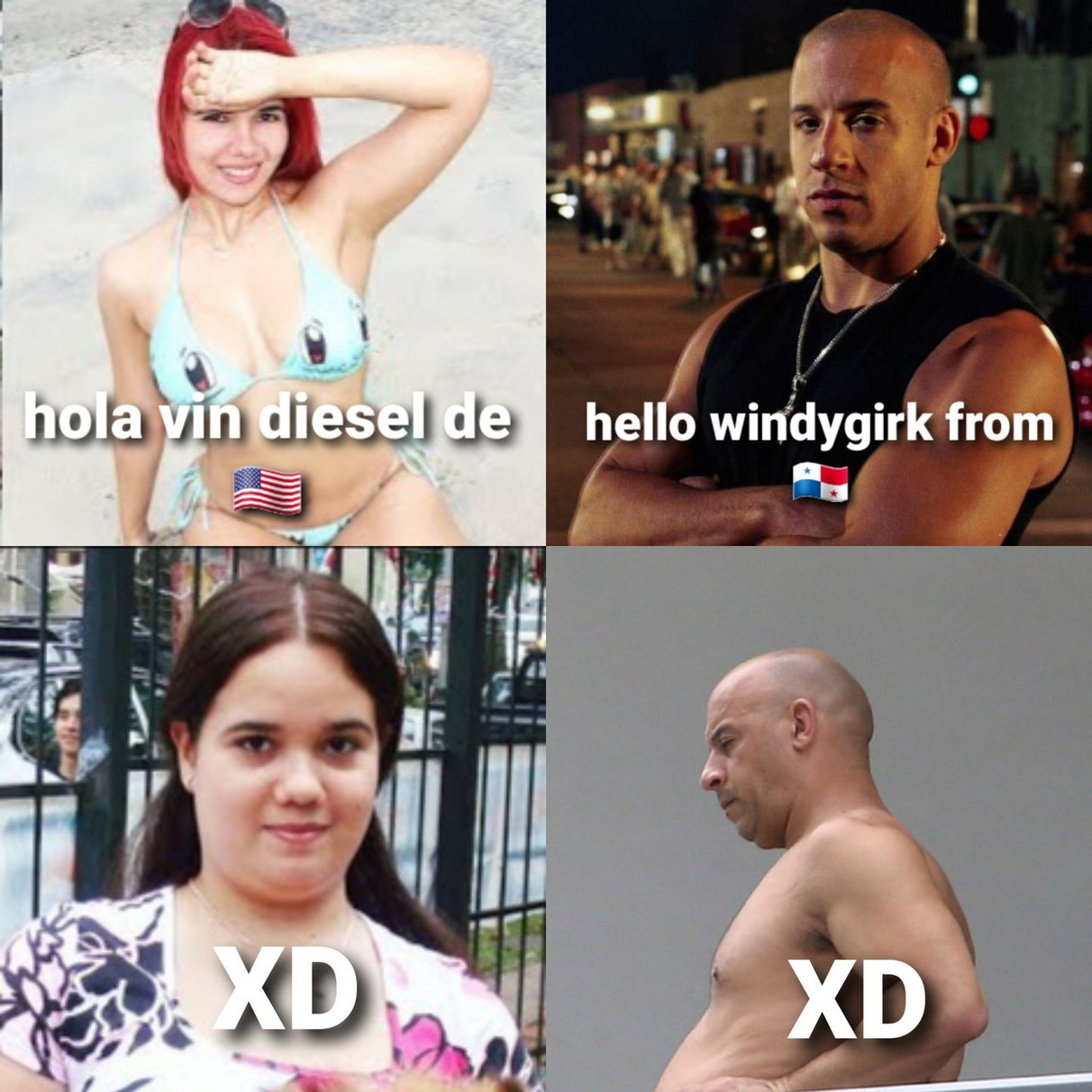This meme is divided into four equal sections, each containing a photograph with text. In the top left quadrant, there's an image of a girl with red hair, wearing a bikini decorated with the Pokémon Squirtle. She has sunglasses perched on her head and stands against an American flag background. The text above her reads, "Ola Vindiceldi." 

Next to her, in the top right, is a photo of Vin Diesel from the "Fast and Furious" series. He wears a black tank top with a bar in the background, staring directly into the camera. The text here says, "Ola, windy girl from" with a Panamanian flag below.

In the bottom left segment, the same red-haired girl appears again, now visibly heavier, standing against a city street with a fence behind her. The text simply reads "XD."

In the bottom right, Vin Diesel is shirtless, showing a noticeable belly, and looks off to the side against a gray background. Above him, the text also says "XD," indicating laughter or amusement. 

The meme humorously contrasts the fit and less fit appearances of both characters while using playful text and national flags to add context to the visual joke.